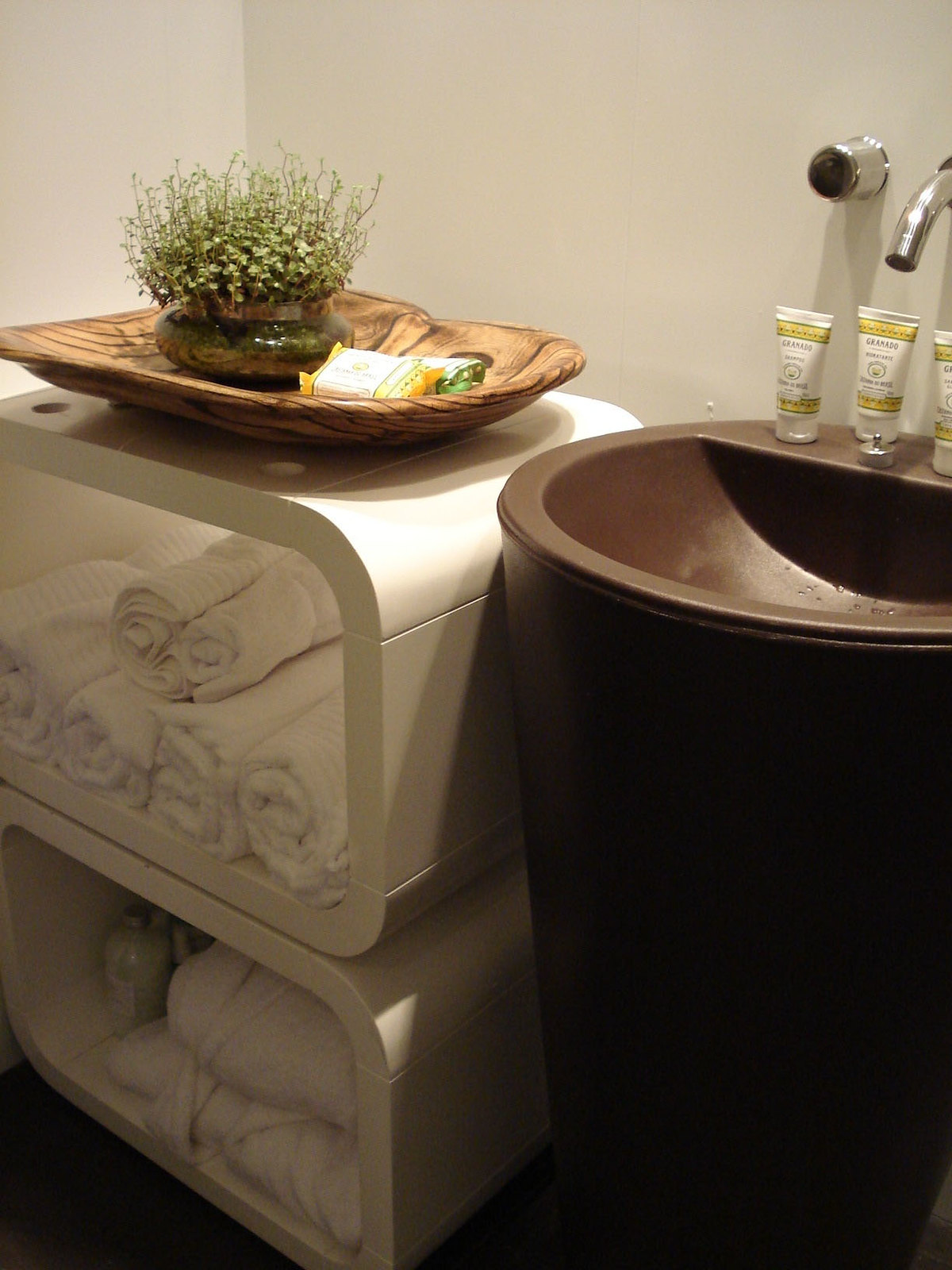The image captures a tastefully decorated bathroom with a cozy, hotel-like ambiance. On the right side of the bathroom, there is a brown sink, adorned with three elegant lotion bottles that are white with gold accents. To the left of the sink, there is a rustic wooden holder, serving as a wash bin, which houses a lush plant with broad green leaves. Nearby, a bar of soap rests in its packaging, alongside what appear to be shampoo bottles. At the bottom left of the scene, there are several white, open rectangular containers filled with neatly folded white towels, while additional bottled amenities can be seen below. The overall setting is indoors, exuding warmth and comfort.